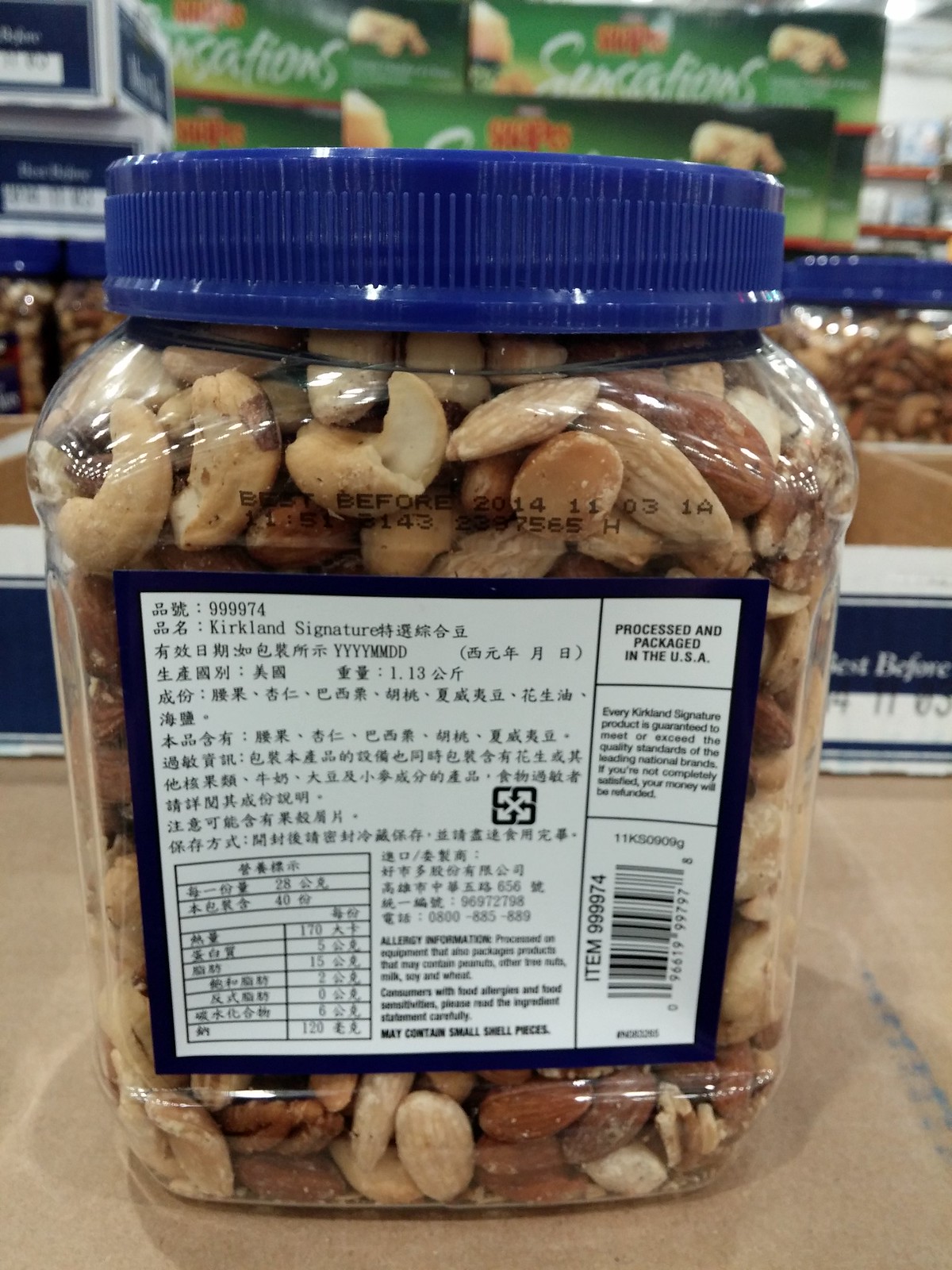This color photograph features a clear plastic container filled with mixed nuts. The container is topped with a blue plastic lid. The image is taken in close-up, focusing on the back label of the container. The label is predominantly white with black text, most of which is written in kanji characters. 

Key details on the label include the number "999974" and the "Kirkland Signature" logo. Additionally, there is visible allergen information indicating that the product is processed on equipment that also handles other products, and it warns that the nuts may contain small shell pieces. Another part of the label states that the nuts are processed and packaged in the USA. 

The label further assures customers that every Kirkland Signature product is guaranteed to meet or exceed the quality standards of leading national brands, offering a money-back guarantee if customers are not completely satisfied. The transparent container reveals an assortment of brown nuts inside.